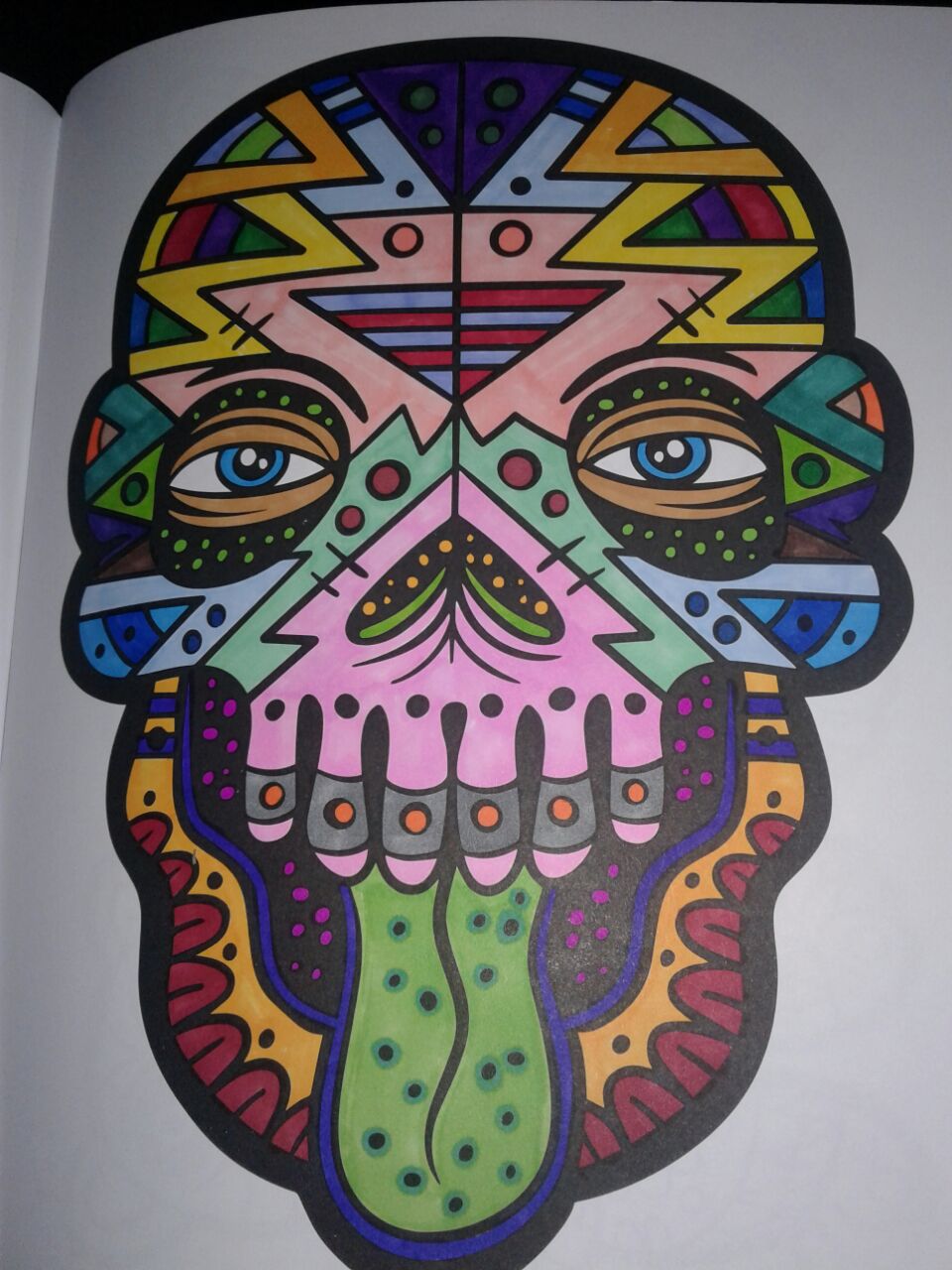This image portrays a vibrantly colored African mask prominently displayed on a white page within a book. The book's binding is visible just at the upper left center fold, where the background transitions from pure black to white. The mask dominates the center of the photo, beginning with a purple triangle adorned with green dots at the top. The mask's design includes orange and yellow zigzag lines resembling a 'W' or 'V' shape that extend along the sides of its skull-like form. 

Intricate details define the mask’s facial features: the eyes are strikingly blue with black pupils encircled by white dots, and the nose is depicted as a black 'V' with orange spots, giving it a butterfly-like appearance. A vibrant green tongue, lined with thin black squiggles and dotted with blue, emerges toward the mask's lower center. The teeth are represented by red arch-shaped patterns, above which yellow sections with black dots create additional texture.

Overall, the head is an interplay of geometric shapes and dynamic lightning bolt patterns in colors that span the spectrum—pinks, blues, greens, yellows, oranges, and reds. The fusion of these striking colors and patterns gives the mask its lively and mesmerizing appearance.